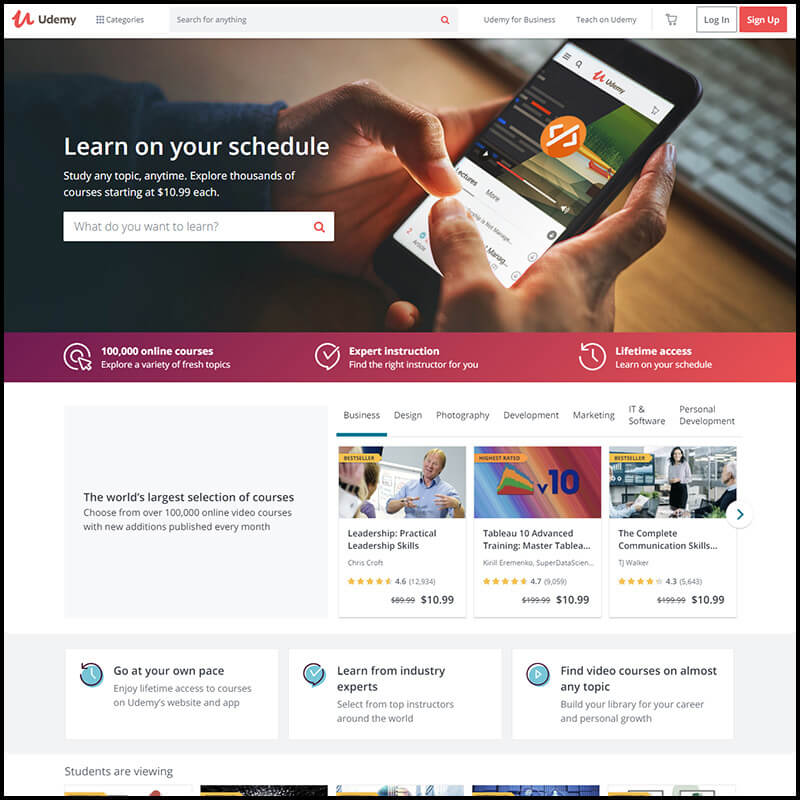This is a screenshot of the Udemy website. The header is white and starts with a pink, cursive "U" logo on the left side. Adjacent to the logo is the brand name "Udemy" in dark gray text, with a capital "U" followed by lowercase letters. There's some negative space, followed by a 3x3 grid of light gray dots. Next to the grid, "Categories" is written in light gray text. A light gray search bar sits to the right, containing medium gray placeholder text that reads "Search for anything" and a pink magnifying glass icon on the right end.

Continuing to the right, after more negative space, is "Udemy for Business" in light gray text. Following that is "Teach on Udemy," then a vertical light gray separator line. To the right of the separator, there is a medium gray shopping cart icon. Next comes a white button with a thin medium gray outline, featuring "Login" in medium gray text. Finally, a pink button with white text labeled "Sign Up" rounds out the header elements.

Beneath the header, a photograph fills the background of the website. It showcases a person's arms extending from the right side, both hands holding a cell phone with a black bezel. The phone screen displays a website with a white background and an orange circle at the top center. The circle features a white left-pointing arrow, a white right-pointing arrow, and a white slash between them. The left side of the image darkens, overlaid with centered white text that reads "Learn on your schedule." Below this text, two lines of smaller white text are also noticeable.